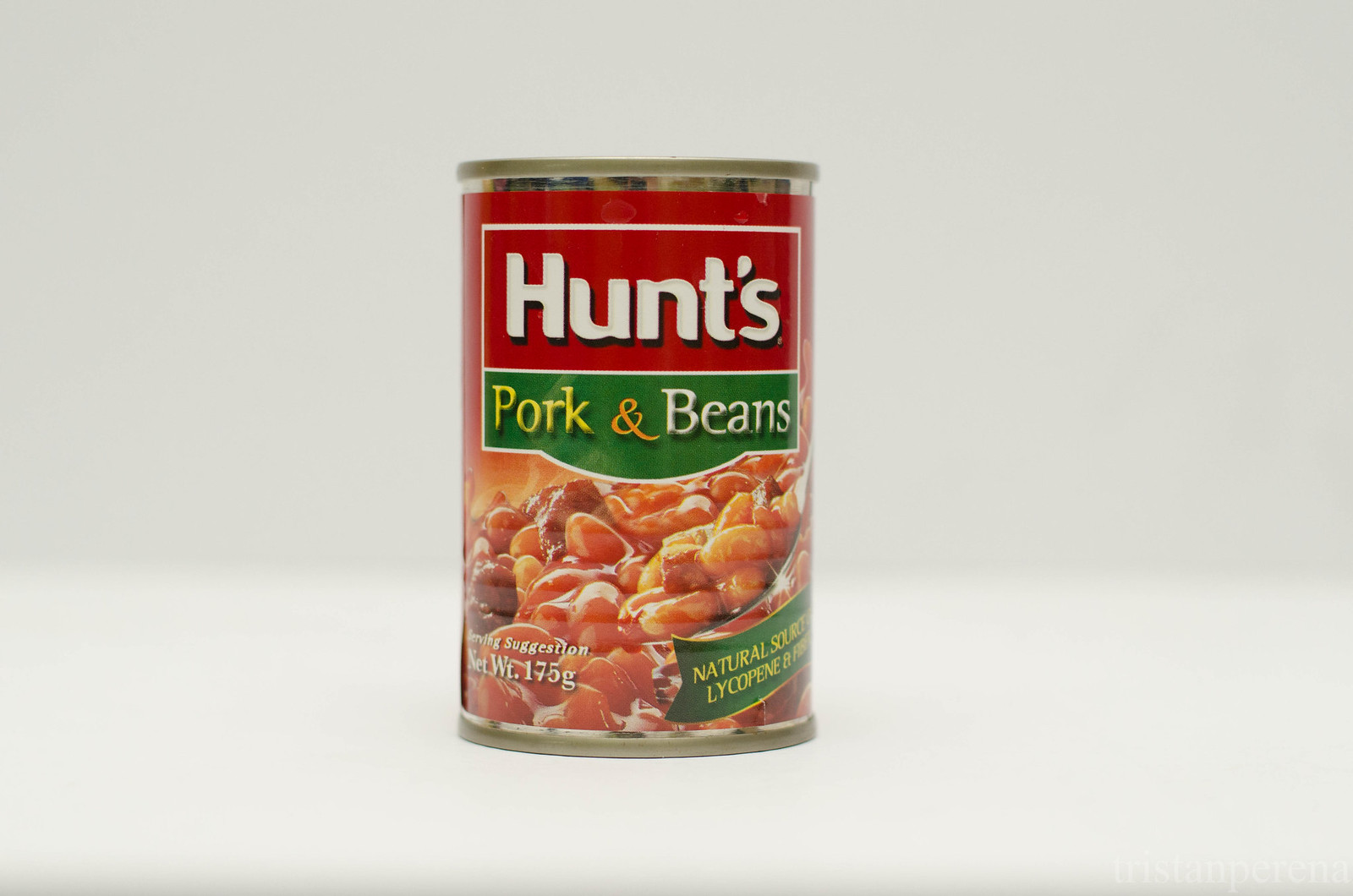This image showcases a Hunts brand can of pork and beans, prominently placed against a stark white background. The can features a vibrant red logo with the words "Pork & Beans" situated in a green section towards the bottom. An appetizing image depicting the pork and beans is displayed prominently on the label, alongside the text "Serving Suggestion." Directly below the image, the net weight is specified as 175 grams. Additionally, a note on the side of the can mentions that it is a "Natural Source of Lycopene," though part of this text appears to be cut off. Notably, the can appears to lack a shadow at its base, giving it a seemingly photoshopped appearance against the pristine white backdrop.